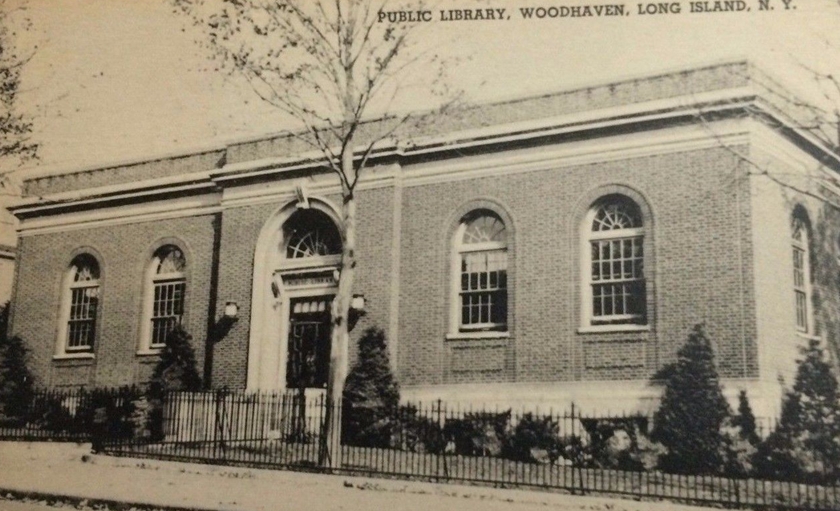This sepia-colored vintage postcard captures a detailed exterior view of the Public Library, Woodhaven, Long Island, New York. The single-story brick building features a grand entranceway with a black door centered between two windows on each side. Above the door, a white stripe runs horizontally across the façade, adding a subtle contrast to the brickwork. The library is framed by a black iron fence that extends along the entire length of the building, leading to a sidewalk in front. In front of the building stands a single leafless tree, indicative of either spring, fall, or winter, alongside four small, conical trees resembling Christmas trees. The black lettering at the top of the building clearly identifies it as the Public Library.